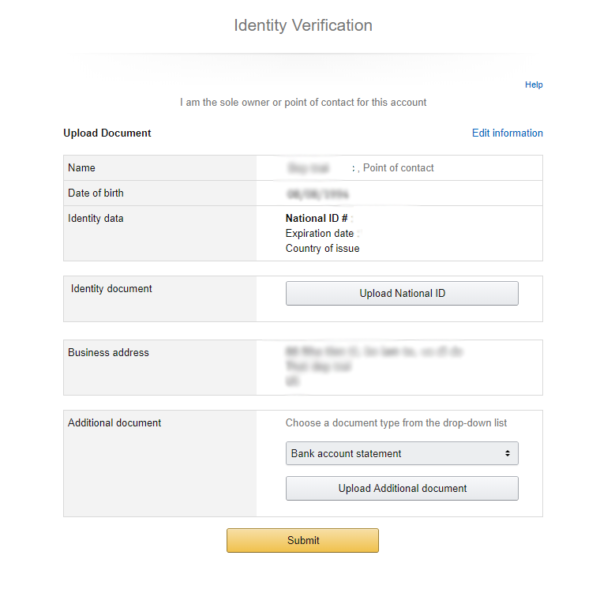This is a detailed screenshot of an ID verification page. At the top, there is a header titled "Identity Verification." Directly beneath this header is a directive stating, "Find the sole owner or point of contact for this account," accompanied by a blue "Help" button positioned to the right.

The section below this can be segmented into four main tables:
1. **Upload Document and Edit Information**: On the left side, there is an "Upload Document" button, while on the right side, there is an "Edit Information" button both in blue.
2. **Personal Information**: This table lists "Name," "Date of Birth," and "Identity Data" on the left side. Below, it specifies "Identity Documents" with an accompanying "Upload National ID" button on the right, which is a gray rectangle.
3. **Business Address**: The left side of this table is labeled "Business Address," with the right side of the information blurred out for privacy.
4. **Additional Documents**: The left side is labeled "Additional Document," with instructions to "choose a document type from the dropdown list." Below, there is a dropdown that currently displays "Bank Account Statement," followed by an "Upload Additional Document" button underneath.

This image provides an organized and structured layout for completing ID verification through various document submissions and edits.